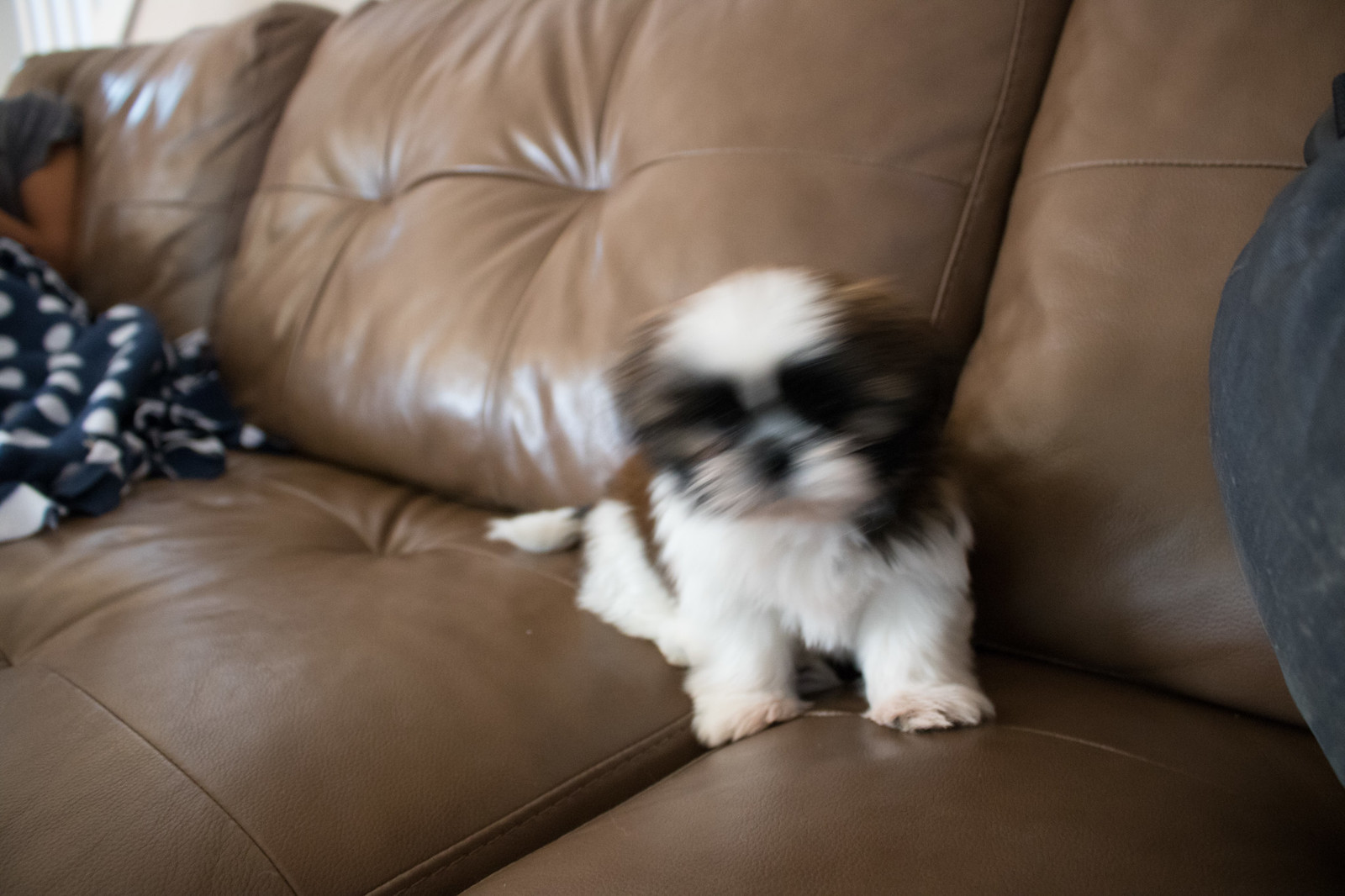This indoor photo captures a small, cute puppy, likely a Shih Tzu, with distinctive dark markings around its eyes and ears, accented with white fur on its forehead, muzzle, and chest, along with some brown patches on its back. The image is slightly blurry, giving a sense of motion, as the puppy nestles between the cushions of a large, plush, brown leather sofa. The couch appears comfortable and expansive, showcasing at least three sections of cushions. To the left of the frame, a person wrapped in a navy blue blanket with white polka dots is partially visible, wearing a dark gray t-shirt. In the background, to the top left, there are white stair railings, hinting at a cozy, homely setting.